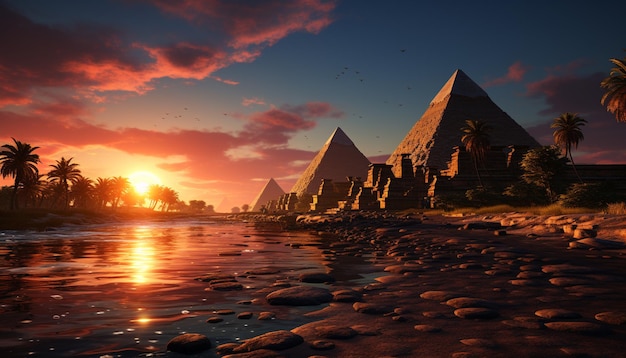This highly detailed image, potentially an AI-generated representation of Egypt during a vibrant sunset, showcases the ancient landscape in hyper-realistic colors. Dominating the scene are the three great pyramids positioned toward the right, with one nearer to the horizon appearing smaller and the other two more prominently displayed, revealing intricate brick details. At the base of the pyramids, a pile of unused stones or possible ruins is visible, adding to the historical essence. In the foreground, a bare riverbank leads to the presumed Nile River, reflecting a deep blue with hints of red, interspersed with water rocks. The river wraps from the center-left to the right of the image. The left horizon is adorned with a line of palm trees through which the setting sun casts a brilliant orange glow, tinged with red and pink hues, onto the water. Additional palm trees stand to the right of the image, dotting the riverbank. The sky transitions dramatically from the left to right, starting with hues of red and orange cloud cover to a deeper cerulean blue beset with darker gray and purple clouds. Black birds can be seen gliding across the dusky sky, adding a sense of movement to this picturesque landscape.